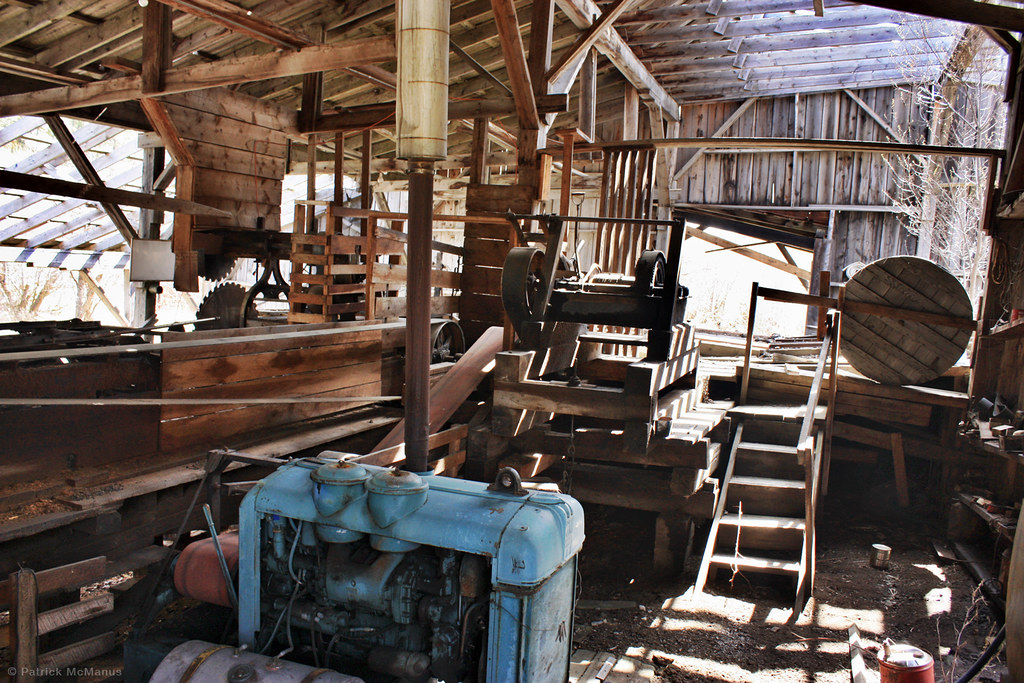This image captures the interior of an old, dilapidated barn primarily constructed from wood. Sunlight filters through gaps in the roof and walls, illuminating dust particles in the air and highlighting the structure's aged, weatherworn beams and rafters. Prominently featured in the foreground is a blue, antique metal engine with a pipe extending from its top, possibly part of a defunct conveyor system used for timber processing. Adjacent to it, on the left, are two large, log-cutting saws, further suggesting the barn's former use as a timber mill. Towards the back, a decrepit wooden ladder leans precariously, and additional wooden structures and barrels clutter the scene, each bearing the unmistakable marks of time and neglect. The sun casts long shadows through the barn, mostly from the top right corner, creating a stark contrast against the light brown wooden surfaces. On the bottom right, a ladder leads to a potential second level, and nearby, a circular table lies on its side, adding to the sense of abandonment and disrepair.